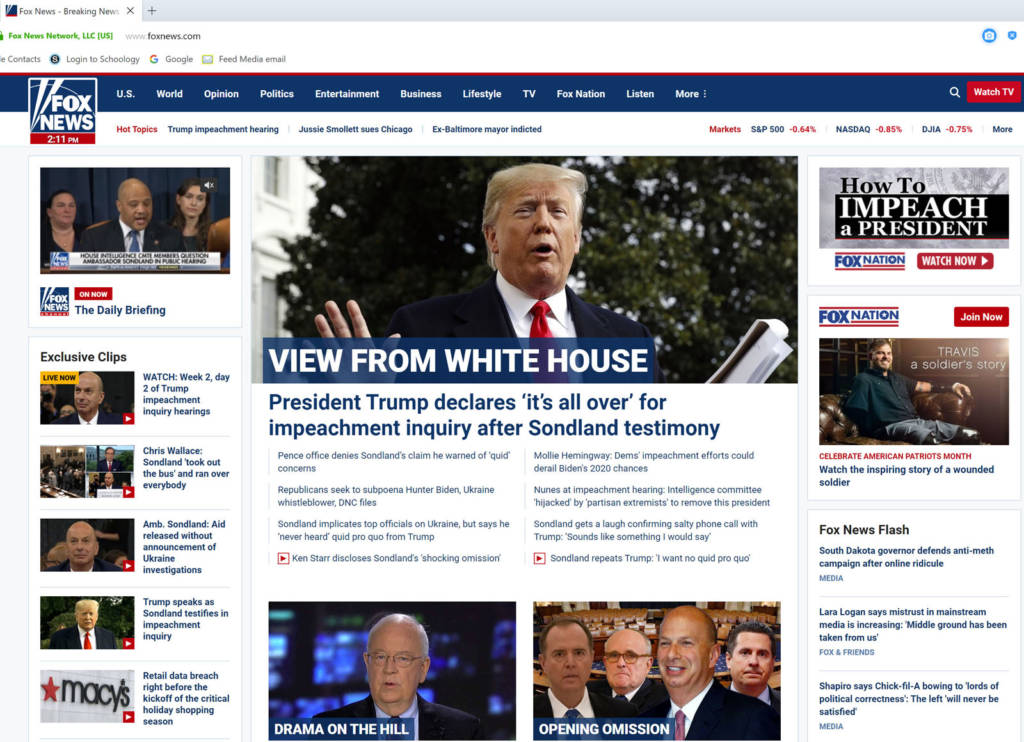Here is the cleaned-up and detailed descriptive caption:

---

This screenshot captures the homepage of the Fox News website. In the upper left-hand corner, an open browser tab clearly indicates "Fox News - Breaking News." Directly below, the website's address is displayed as "Fox News Network LLC, www.foxnews.com." Accessible links for logging into Schoology, Google, and Feed Media Email are situated nearby. 

At the top of the page, a blue banner reads "Fox News 2 11 p.m.," underlined by a navigational menu with clickable categories including US, World, Opinion, Politics, Entertainment, Business, Lifestyle, TV, Fox Nation, Listen, and More. 

Highlighted hot topics draw attention in a separate section, listing "Trump Impeachment Hearing," "Jussie Smollett Sues Chicago," and "Ex-Baltimore Mayor Indicted." 

Scrolling further reveals several headlines: 
- "View from the White House: President Trump declares it's all over for impeachment inquiry after Sondland testimony."
- "Drama on the Hill: An opening omission."

On the right side, additional stories include:
- "Watch the inspiring story of the wounded soldier."
- "Fox News Flash: South Dakota governor ends anti-meth campaign after online ridicule."
- Laura Logan's statement on "mistrust in mainstream media's increasing, middle ground has been taken from us."
- Ben Shapiro's critical commentary: "A Chick-fil-A bullying to lords of political correctness. The left will never be satisfied."